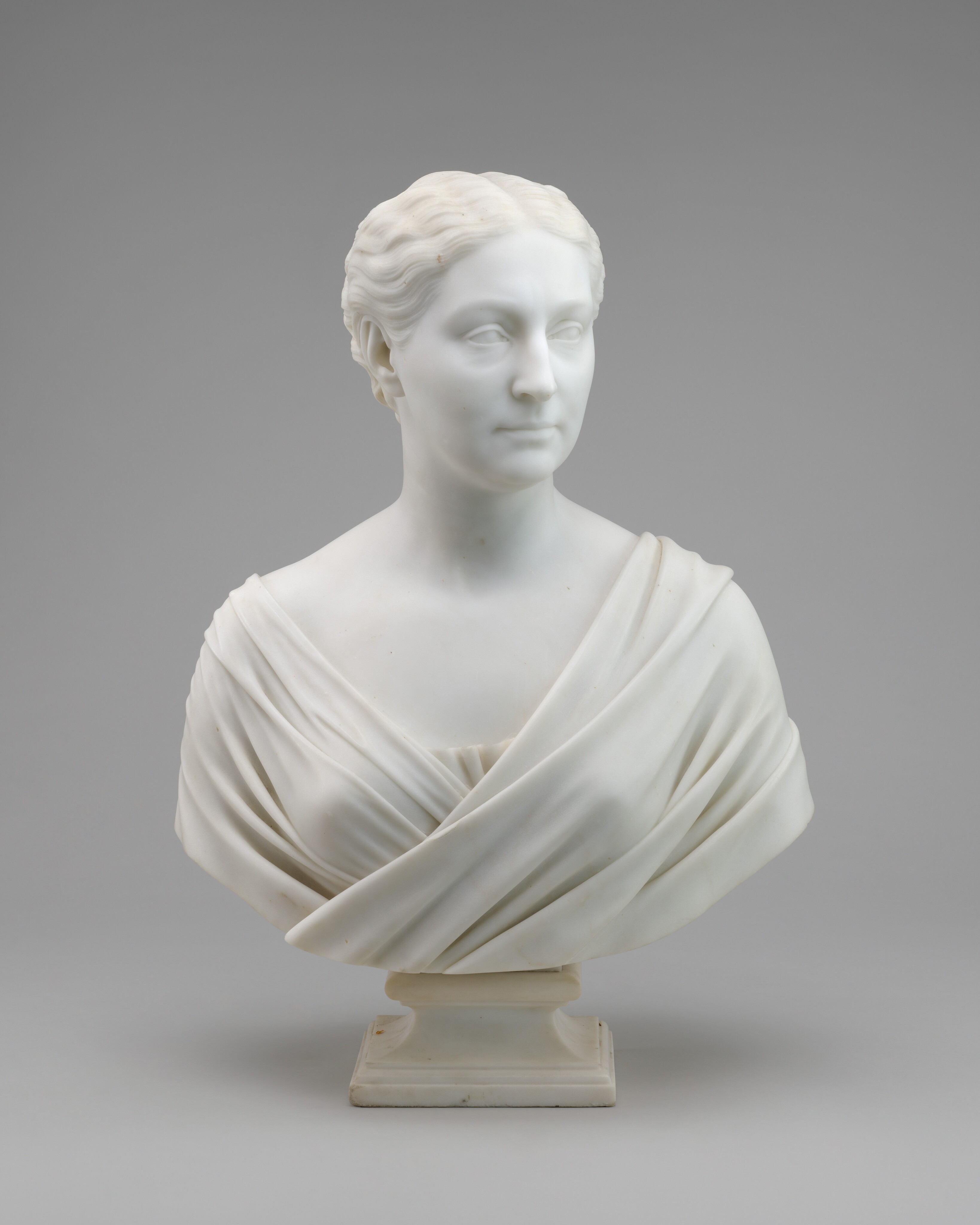This is a detailed colour photograph of a Greco-Roman inspired marble bust of a female figure, placed prominently on a sculpted pedestal against a neutral grey backdrop. The pedestal is square-shaped with multiple lips around its base, tapering inward to support the artwork. The sculpture itself, an off-white to slightly cream colour, depicts the head and shoulders of the woman, dressed in a finely detailed robe. The robe features intricate pleats and overlaps on her chest, with the left side draping over the right. The bust is cut off below the shoulders, lacking arms, and the robe's neckline is smooth.

The female figure's head is turned slightly to the left, creating a sense of contemplation or focus on something in the distance. Her facial features, including a neutral expression with a subtle hint of a smirk, mouth, nose, and featureless eyeballs, are masterfully carved, emphasizing the lack of pupils, which adds a haunting quality to her gaze. Only her right ear is visible due to the head's turn, and her wavy hair is centrally parted and tucked behind her ears, extending just slightly behind her head.

The pedestal, slightly yellowed compared to the sculpture, adds an aged elegance to the display, enhancing the timeless beauty of the bust. This photograph captures the essence of the artwork with deliberate emphasis on the sculpture’s fine details and textured quality, presenting it as a timeless piece of art showcased out of context for visual appreciation.